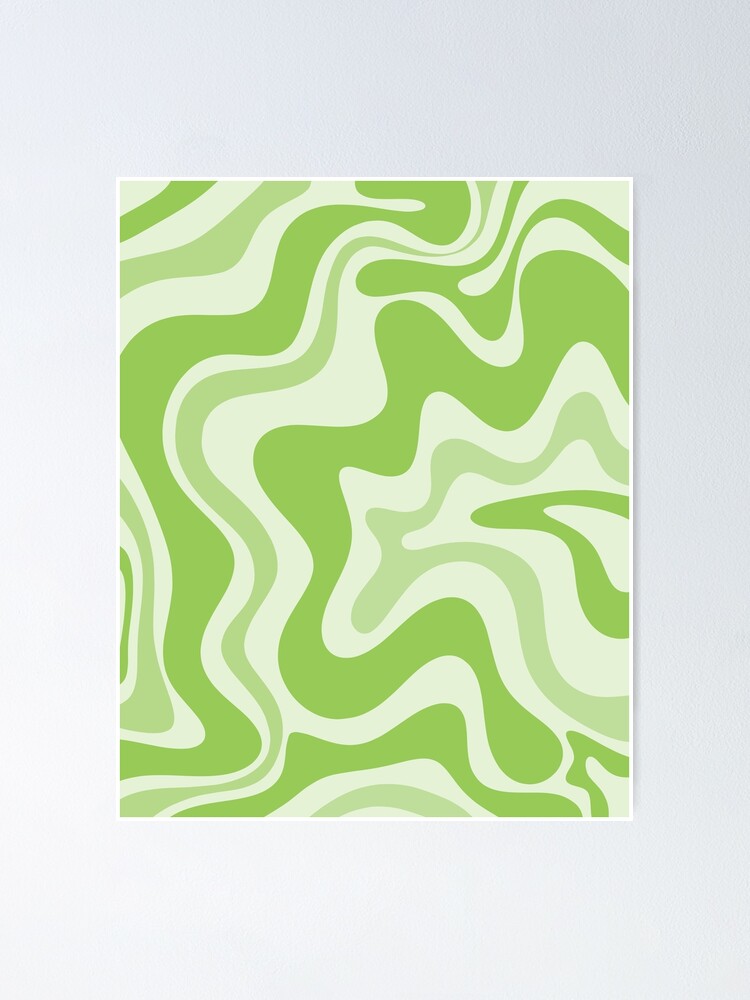This image is an abstract painting on a vertically oriented canvas with a fine white frame. The background is a gradient that transitions from a grayish-blue at the top to white at the bottom and left side. The painting itself features a flowing, curvilinear pattern reminiscent of a psychedelic or wood grain design. At the center, there is a snake-like form composed of alternating wavy lines in lime green, light lime green, and white. These lines create a sense of movement as they extend from the right side of the image, curve down to the left, and back to the right, with the pattern repeating across the canvas. The colors—lime green, light lime green, and white—interact fluidly, giving the impression of melting or swirling lines, which creates a visually dynamic and mesmerizing effect, gradually becoming less tightly woven toward the right side of the painting.